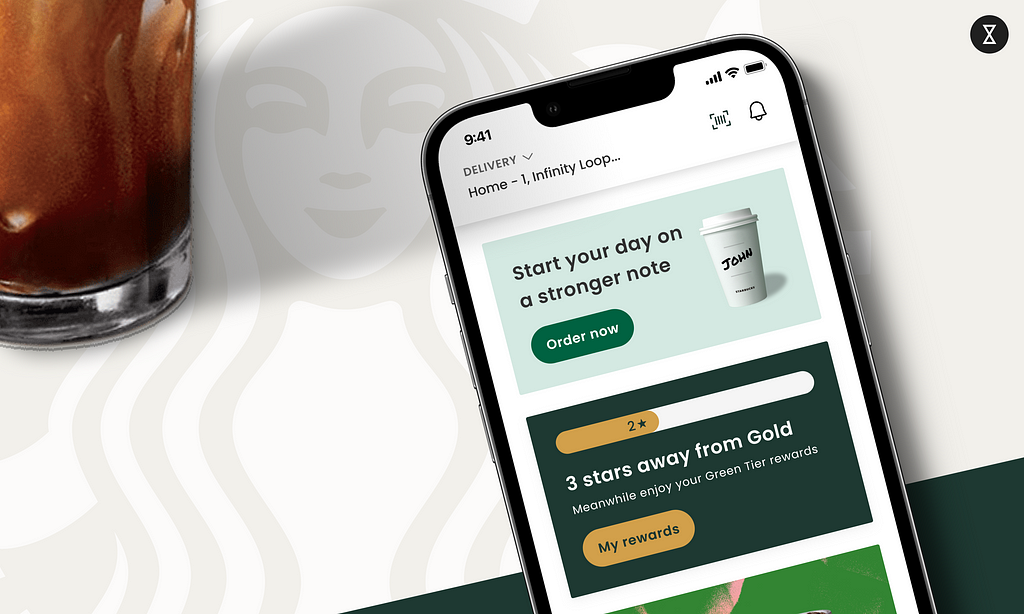A detailed image caption could be:

"In this vibrant scene captured at a Starbucks, a smartphone rests atop a table distinguished by its characteristic Starbucks mermaid logo framed in green. A glass cup containing a beverage accompanies the phone, its positioning creating an intriguing visual angle. The smartphone's screen displays the time as 9:41, with a full battery and a delivery notification indicating 'Home, One Infinite Loop'. The display features an enticing message, 'Start your day on a stronger note,' accompanied by an image of a Starbucks cup bearing the name 'John' and a prompt to 'Order now', all set against a light mint green background.

Beneath this prompt, a reward tracker in a darker green hue announces, 'Three stars away from Gold,' with a motivational note to enjoy 'Green Tier rewards' in the meantime. Even though the cup in the image appears plain white and lacks visible Starbucks branding, the digital interface continues to reinforce the brand's loyalty program. The bottom section of the phone screen, colored in a deeper green, hints at additional features with the 'My Rewards' button, though details are not clearly visible. This setup subtly suggests a Starbucks enthusiast immersed in the brand's rewarding experience."